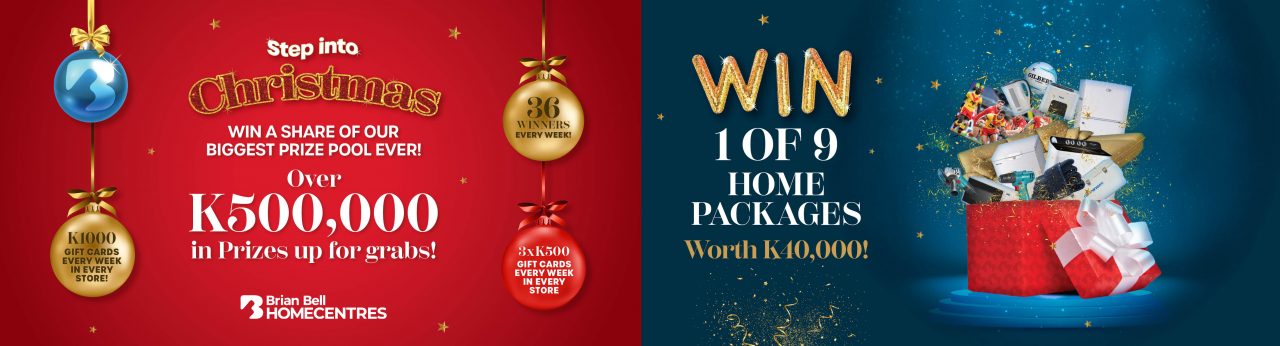The image is a banner composed of two sections: the left side, which is red and adorned with Christmas ornaments, and the right side, which is blue. The left section of the banner features an array of ornaments: a blue one on the upper left, a gold one beneath it, and on the right side, a gold ornament with a red one below it. In the center of this section, the text "Step into Christmas, win a share of our biggest prize pool ever" is prominently displayed, with the word "Christmas" in bold red text with a gold outline and the remaining text in white. Below this, the banner announces, "Over K 500,000 in prizes up for grabs," followed by "Brian Bell Home Centers."

The right section of the banner highlights a promotional offer. The word "Win" is written in striking gold text, followed by "one of nine home packages" in white, and "worth K 40,000" in gold text. The visual centerpiece is a red gift box with a white bow, its lid tilted open to reveal a variety of home products spilling out, including a drill and several boxes.